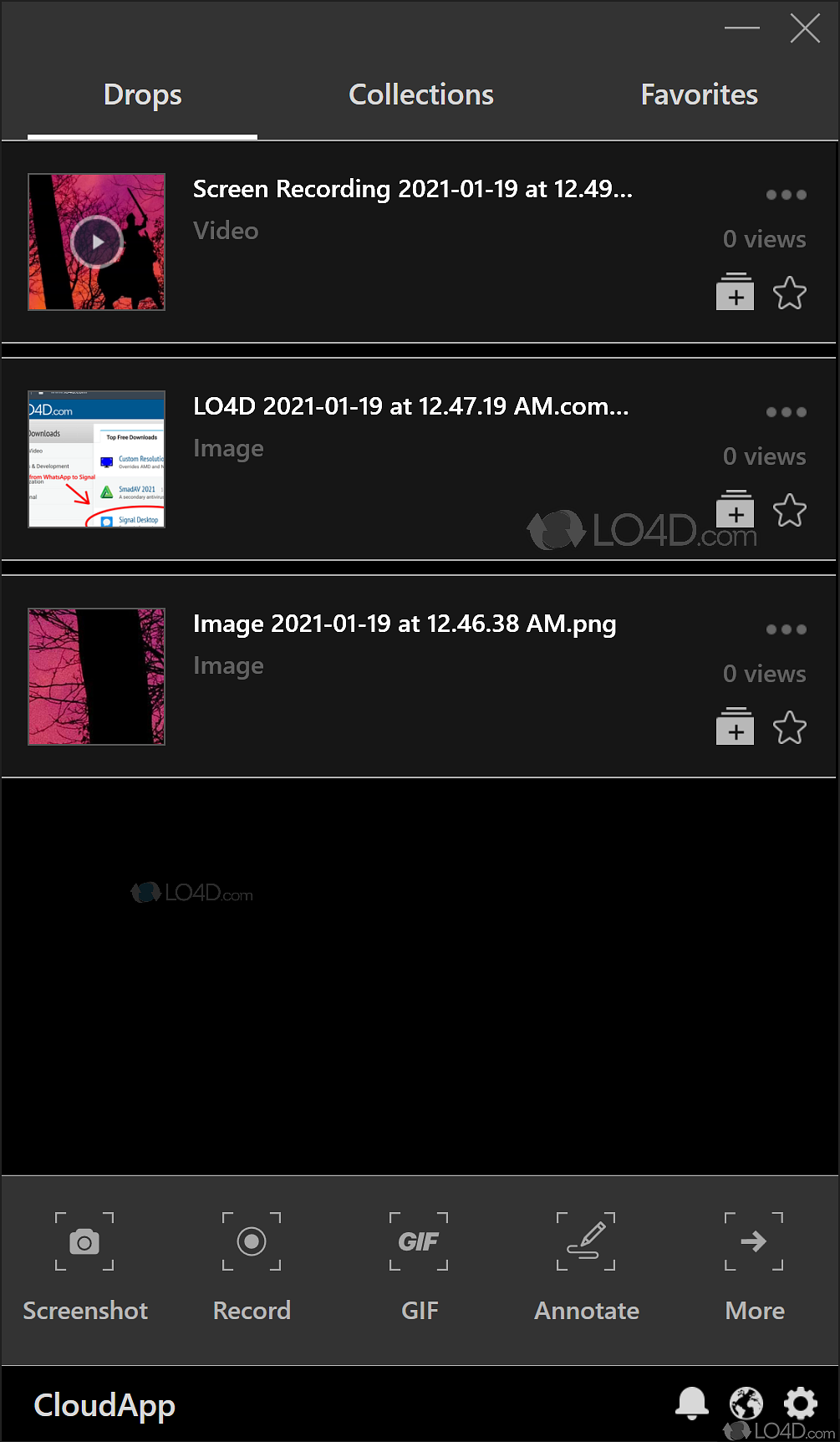This image is a screenshot of an app called Cloud App. The background of the screenshot is entirely black. At the top of the screen, there is a header section that is slightly lighter than the background. In the top-right corner of the header are an X button and a minimize button. The header also contains three titles in white text: "Drops" on the left, "Collections" in the center, and "Favorites" on the right. These titles indicate the different sections within the app.

Below the header, the main part of the image displays three different files. The first file is a screen recording titled "Screen Recording," created on January 19, 2021, at 12:49 (the specific time of day is unclear). It features a thumbnail on the left and a menu on the right, indicating that the file has zero views. Below this information, there are options to download the file and to add it to favorites, represented by a star icon.

The second file is named "LO4D" and was created on January 19, 2021, at 12:47:19 (again, the specific time of day is not clear). Like the first file, it includes a thumbnail, a zero views indicator, and options to download and add to favorites.

The third file is an image with the filename "12.46.38am.png," created on the same date at 12:46:38. This file also shows zero views and includes the download and favorite options.

At the bottom of the image is another menu with five options, each accompanied by an icon: "Screenshot," "Record," "GIF," "Annotate," and "More." Finally, a thin footer at the very bottom of the image reads "Cloud App" on the left and displays three icons on the right: a notification icon, an unknown icon, and a settings icon.